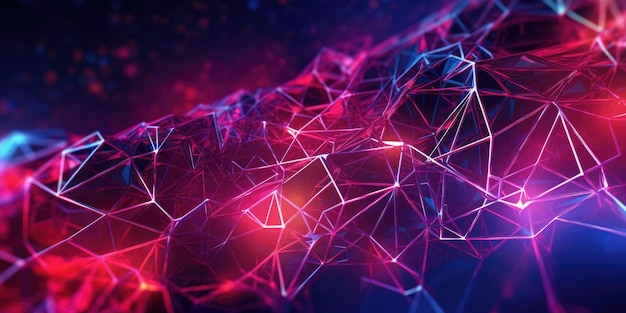The rectangular image is a vibrant and abstract digital artwork composed of interconnected geometric shapes, resembling a web or mesh. The design features segments that evoke the structure of a broken geodesic dome, but arranged in a strand, possibly alluding to a nerve structure or DNA. The color palette is rich and vivid, dominated by reds, purples, blues, and pinks, with sharp white highlights adding definition and depth to the composition. The main focused section stands out sharply against a darker, blurred background, giving the impression of an expansive, intricate network. The image is illuminated in certain areas, creating a glowing effect that enhances its striking appearance against the dark background.